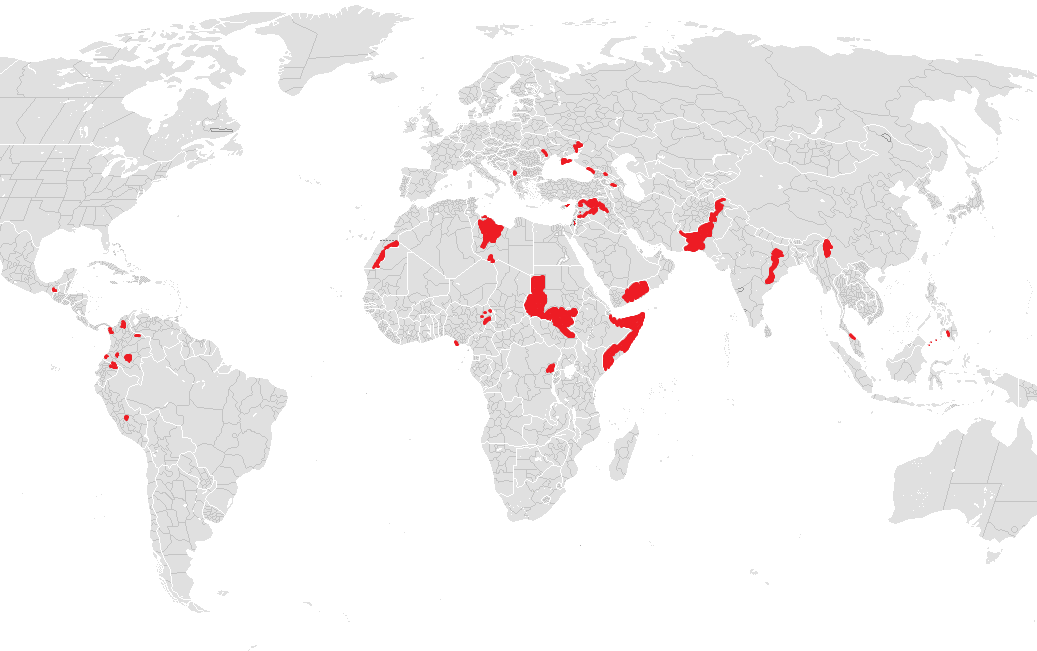The image is a detailed map of the world where the landmasses are depicted in a gray color and the oceans are rendered in white. Delineations between different countries, states, and continents are marked with fine black lines. The map features parts of the world such as half of the United States and Canada up to Texas, and complete views of Africa, Europe, Asia, Australia, and New Zealand. Numerous regions are highlighted in bright red, predominantly situated across Africa, particularly in the center and top left corner, as well as Central America, eastern Europe, South America, the Middle East, and the area surrounding India. The specific significance of the red areas remains unclear, as no legend is provided.